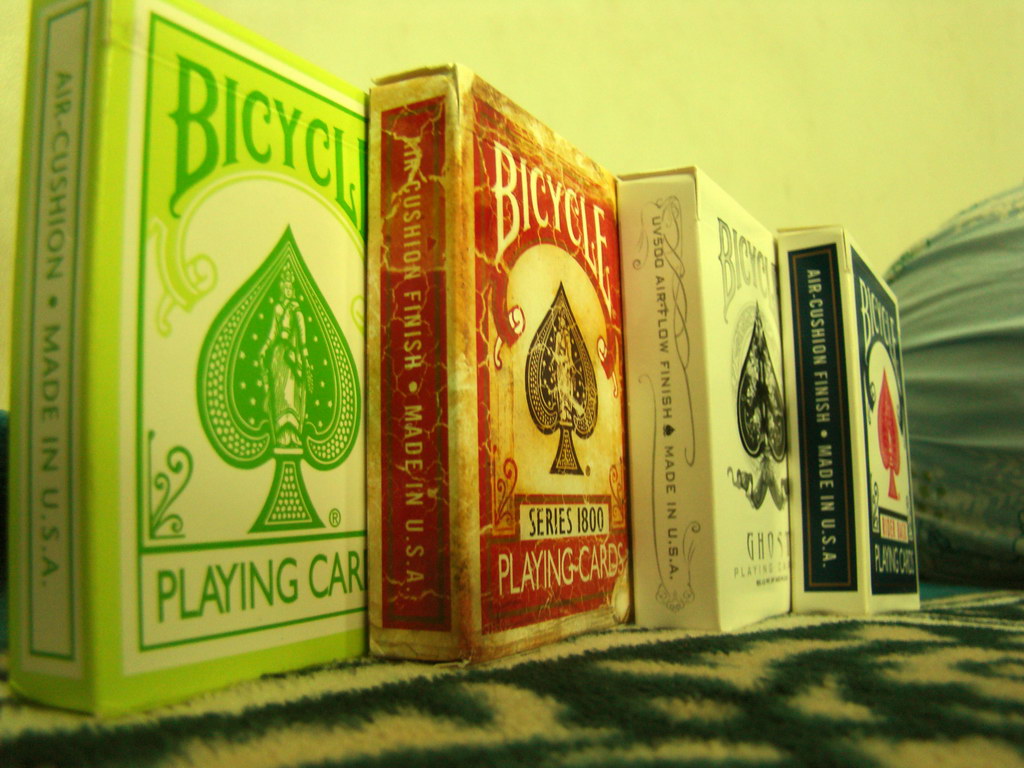A vibrant, indoor landscape photograph showcases four packs of Bicycle playing cards arranged diagonally from the left side of the frame to the right. The closest pack on the left features a striking green edge and an off-white background, with a partially visible "Bicycle" logo. The lower text is cut off, showing only "Car" from "Playing Cards." The front design displays a spade symbol adorned with shades of green, white dots, and a seated royal figure. 

Next in line, a slightly worn pack stands in front, displaying a dominant red tone. The cardboard shows signs of wear with visible creases and cracks. Behind it, the third pack presents a sleek design with a predominantly white background accented by black detailing. 

Furthest away, the final pack contrasts sharply with a predominantly black background highlighted by white edges, featuring a bold red spade emblem on the front. All packs collectively represent various artistic iterations of the renowned Bicycle brand playing cards.